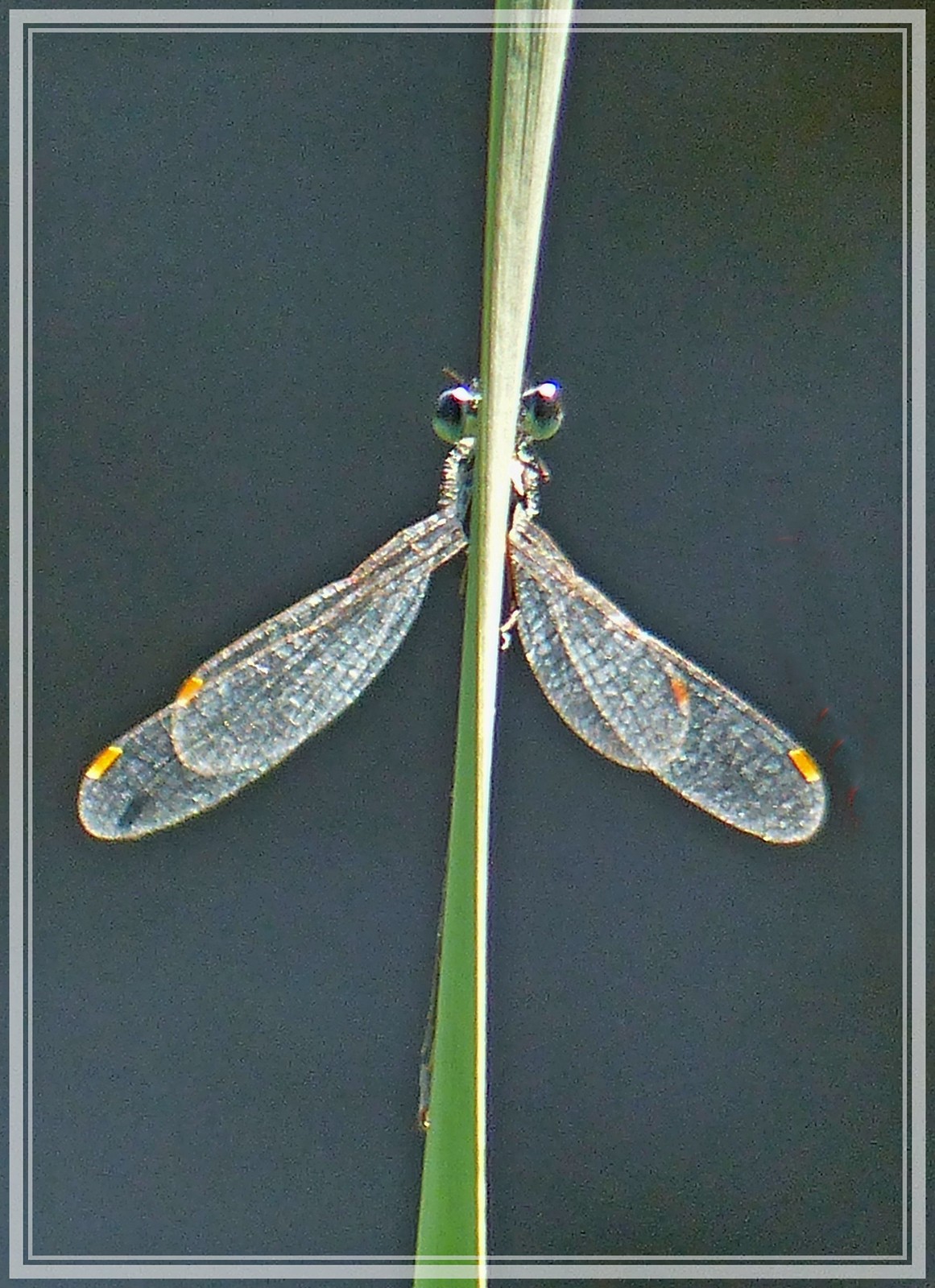This detailed close-up color photograph, in portrait orientation, showcases a dragonfly perched on a tall, vertically oriented blade of grass, which effectively divides the insect into symmetrical halves. The dragonfly, facing the viewer, displays impressive anatomical details. Its large, bulging eyes are iridescent light green on the lower parts and dark gray on the upper parts, with antennae jutting from the top of its head. The wings, near-transparent but not quite, exhibit delicate rectilinear light orange notches near the top edge. One wing appears slightly longer than its counterpart. The body, exhibiting a circular shape with a silvery outline, has a visible little white leg on the right side of the image. The thorax is adorned with hair-like structures that glisten, possibly appearing clear or moist. The dragonfly's partial tail is visible peeking from behind the blade of grass near the bottom. The background features a greenish-gray or dark teal hue, adding contrast and focus to the dragonfly, with the entire image framed elegantly in what appears to be a silver photo frame. The style exemplifies photographic representational realism.